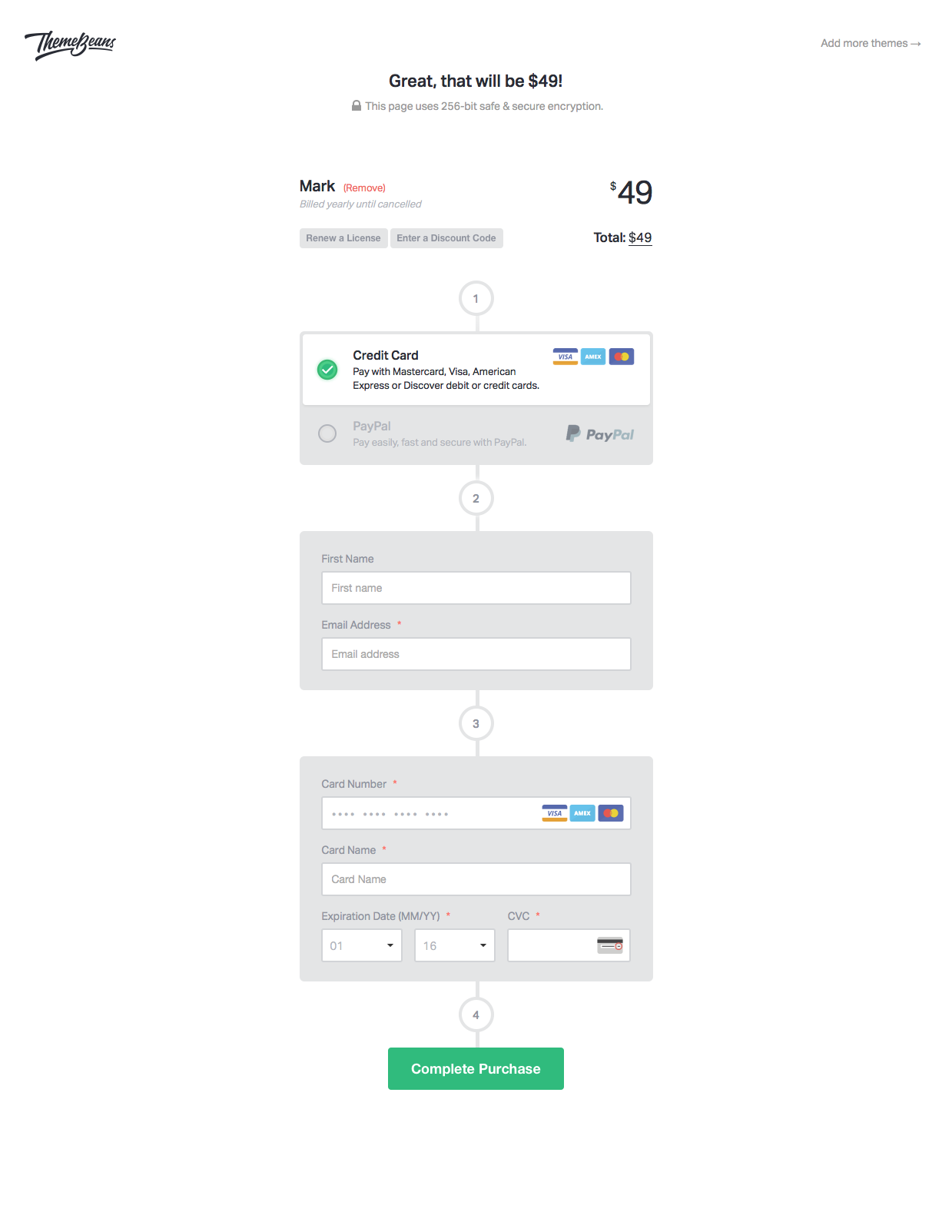The image displays a detailed payment form for purchasing a product or service online. 

In the top left-hand corner, an element is visible, while in the top right corner, there is a button labeled "Add More Themes." Centrally, a message reads, "Great, that will be $49," with a lock symbol and text below stating, "This page uses 256-bit safe and secure encryption."

Further down, an option marked "Mark" is accompanied by red text in parentheses, "Remove." Below this, it indicates "Billed yearly until canceled," followed by two buttons labeled "Renew License" and "Enter Discount Code." Adjacent to these buttons, to the right, it says "$49 in total," reiterating the amount as $49.

The form is divided into several sections:
1. **Payment Method**:
   - "Credit Card" is checked with a green circle, offering payment via MasterCard, Visa, American Express, or Discover debit/credit cards. Underneath are the respective card logos, currently unselected and shaded in gray.
   - "PayPal" is presented as an alternative method, with the text "Pay easily, fast, and secure with PayPal" and the PayPal logo next to it.

2. **Personal Information**:
   - A field to enter your first name and email address, both required.

3. **Card Details**:
   - Fields to input the card number (required), cardholder name (required), expiration date (MM/YYYY, both required), and the CVC code.

4. **Complete Purchase**:
   - A prominently displayed green button labeled "Complete Purchase" to finalize the transaction.

Overall, the image meticulously guides the user through the payment process, emphasizing security, payment options, and the steps necessary to complete the purchase.